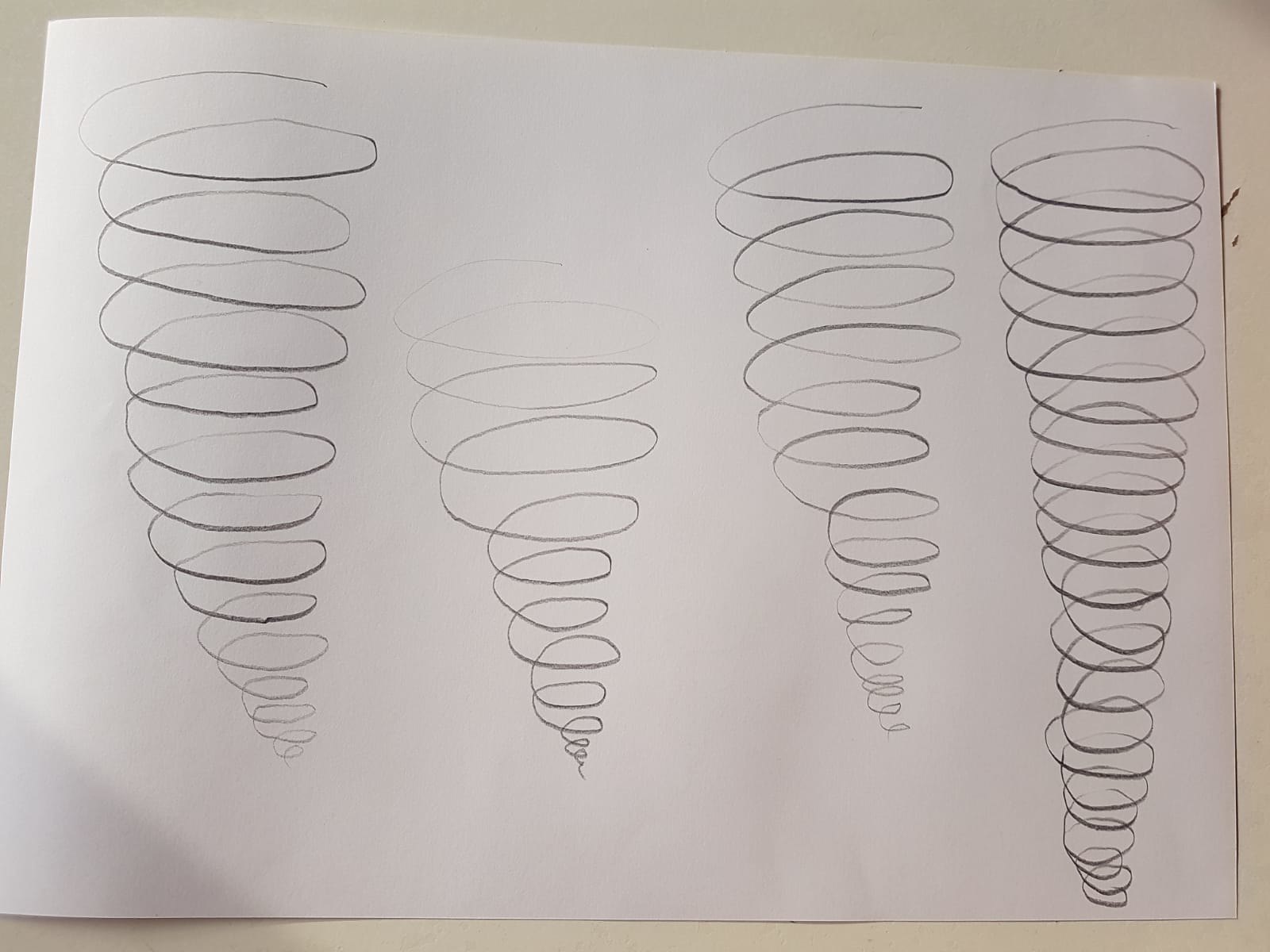The image depicts a piece of white paper with four hand-drawn coil springs arranged in a vertical sequence. Each spring is drawn in black ink, starting with a small, tightly coiled base that expands as it ascends. The first spring at the left edge extends from the bottom of the paper to nearly the top, displaying a transition from smaller to larger coils. Next to it, the second spring starts at a similar base height but reaches only halfway up, with noticeable erasure marks indicating an attempt to remove the top half. The third spring is slightly taller than the second, demonstrating a more defined progression of coil size. Finally, the fourth spring, drawn in a darker, bolder stroke, spans the entire height of the paper, maintaining consistent coil size variation from bottom to top. The paper rests on an off-white table marred with faint, indistinct lines and marks, suggesting wear and usage.